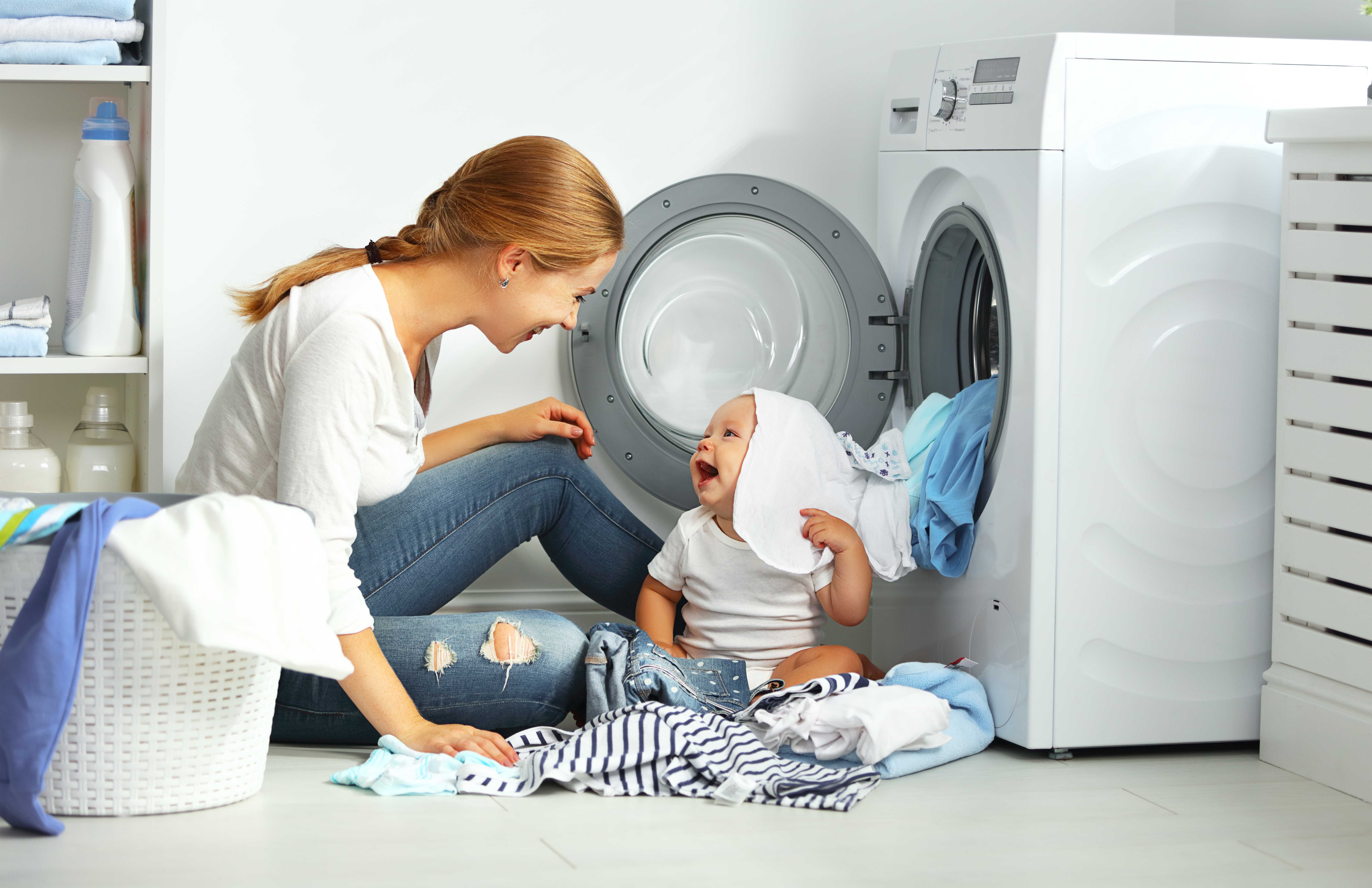The image depicts a lively and intimate moment between a young woman and a baby, seated on a white floor in a laundry room with white walls. The woman, who has ginger-colored hair styled in a single braid down her back, is dressed in a white long-sleeved shirt with the sleeves rolled up and blue denim jeans with ripped thighs just above the knees. She is smiling warmly at the baby, who is looking up at her with a big, open-mouthed smile.

The baby, dressed in a white onesie, sits surrounded by clothes, with a piece of white fabric playfully draped over his head. He appears to be either loading clothes into or taking them out of the open front-loading washing machine. The washing machine and an adjacent hamper are both white, contributing to the overall light and airy atmosphere of the room. 

In the background, a white laundry basket filled with blue and white clothes adds to the scene's realism. Behind them, a white shelf holds various laundry supplies including white containers, bottles, and neatly folded blue and white towels. The shelves also display some laundry soap and detergent, making it clear that the space is fully equipped for laundry tasks. The abundance of white elements—clothing, walls, appliances, and storage—gives the scene a clean and organized feel.